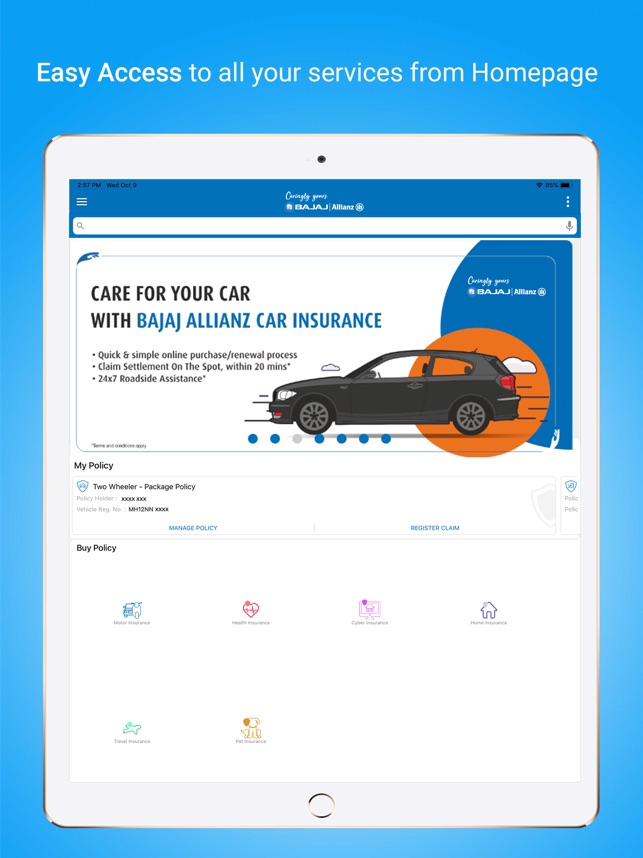In this image, we see a detailed website landing page for an auto insurance service, depicted on a white iPad against a vibrant blue background. Above the tablet, there's a headline that reads: "Easy access to all your services from homepage."

The iPad displays the landing page content, dominated by a banner featuring a sleek black hatchback car. Above the car graphic, the text reads: "Care for your car with Bajaj Allianz Car Insurance." Below this, a slogan touts: "Quick and simple online purchase/renewal process," followed by a promise of "Claim settlement on the spot within 20 minutes" and "24/7 roadside assistance."

Further down the screen, the interface includes a section labeled "My Policy" under which "Two-wheeler Package Policy" is listed. At the bottom of the tablet's display, there is a call-to-action area labeled "Buy Policy," accompanied by clickable icons for user interaction.